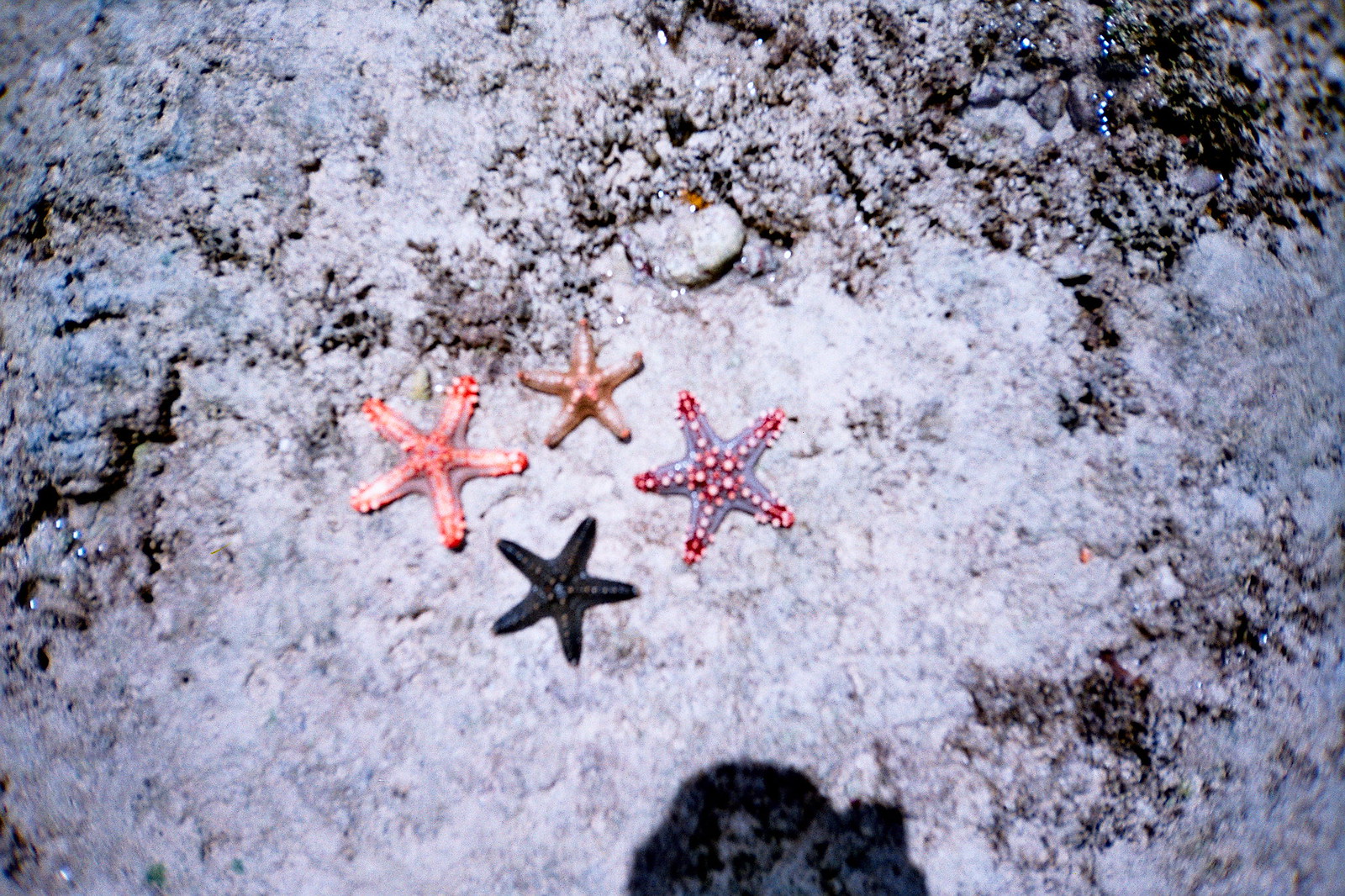This image captures four distinct starfish resting on the white sandy floor of a large body of water, possibly an ocean. Despite their proximity, each starfish showcases a unique design and coloration. On the left, there is a pinkish salmon starfish, while the next one is predominantly red with a striking silver pattern at its center. Moving towards the right, there is a deep jet-black starfish, adding a stark contrast, and lastly, a bluish-black starfish. The sandy floor is interspersed with pale, craggy rocks and coral formations. At the bottom of the image, the shadow of the person taking the photograph is visible, suggesting a bright day. The entire scene is a vibrant display of marine diversity and natural textures.